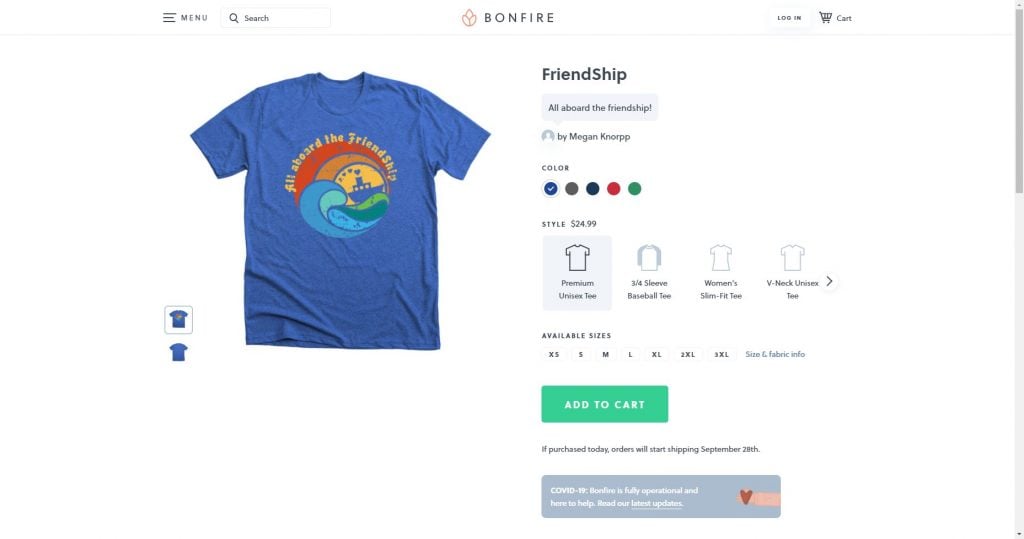This website, called Bonfire, features an intricately designed webpage centered on a t-shirt titled "All Aboard the Friendship." Dominating the center of the page is a vibrant logo that resembles intertwined leaves with an emerging half-circle flame, rendered in shades of orange. To the left, a minimalist navigation menu is displayed with three horizontal lines, followed by a search textbox containing a black magnifying glass icon and the word "Search" aligned to the right. A conspicuous "LOGIN" button in uppercase black letters, a black shopping cart icon, and the word "CART" in black text complete the header setup.

Below, the primary focus is a royal blue t-shirt showcased under the slogan "All Aboard the Friendship." The shirt's design features an enchanting illustration of a boat emitting heart-shaped puffs in place of steam, all encapsulated within a yellow circle. The background includes dynamic blue, aqua, and green waves intertwined with swirling patterns, while the central text is a vibrant yellow.

To the left of the main t-shirt image are icons displaying the front and back views of the shirt. The front view is highlighted, accompanied by the text "FRIENDSHIP" in bold letters. Below this, it states "All Aboard the Friendship" by Megan Can Warp, though no avatar is provided.

A color selection menu is available directly beneath, currently set to royal blue with additional color options including brown, black, red, and green. The shirt is priced at $24.99 for the premium unisex tee, with alternative styles listed such as a three-quarter sleeve baseball tee, women's slim fit tee, and a v-neck unisex tee. A greater-than sign indicates the availability of further style options.

Size options range from extra small to 3XL, and a link is provided for detailed size and fabric information. No size is currently selected. Beneath the size options, a prominent green "ADD TO CART" button is displayed, written in uppercase white letters.

A note just below informs customers that orders placed today will begin shipping on September 28th. Additionally, a gray box at the bottom of the page provides a notification about Bonfire's operational status during COVID-19, along with a link to their latest updates.

Completing the page's design, an arm extends from the right side, holding a heart, symbolizing the community and connection that Bonfire aims to foster through its offerings.